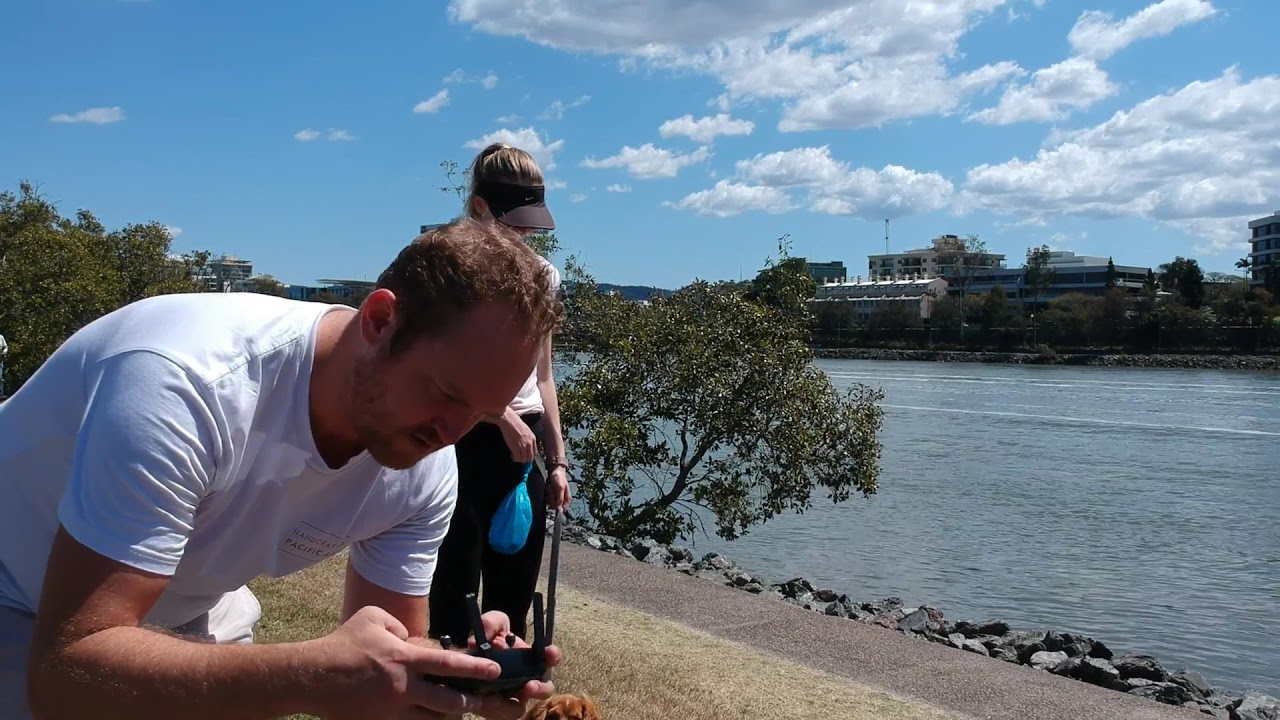In this bright, postcard-style daytime photograph, we see two people and a dog by a tree-lined river, surrounded by buildings with a blue sky and a scattering of white clouds. The foreground features a middle-aged man with brown hair, wearing a white t-shirt, squatting or kneeling as he looks down at a device or equipment in his hand, possibly setting something up like the bottom of a tripod. Beside him stands a woman with a ponytail, dressed in dark pants, a black visor, and a white or light fawn-colored top. She holds a blue plastic bag—potentially containing dog waste—in one hand and appears to have a leash in her other hand, indicating the presence of the small dog whose head is visible. Behind them, across the several-hundred-feet-wide, rock-lined river, there are tree-bordered office buildings or a parking garage, each around four stories high, contributing to the urban day scene. The photograph is a horizontal rectangle fitting the entire scene smoothly within the frame.